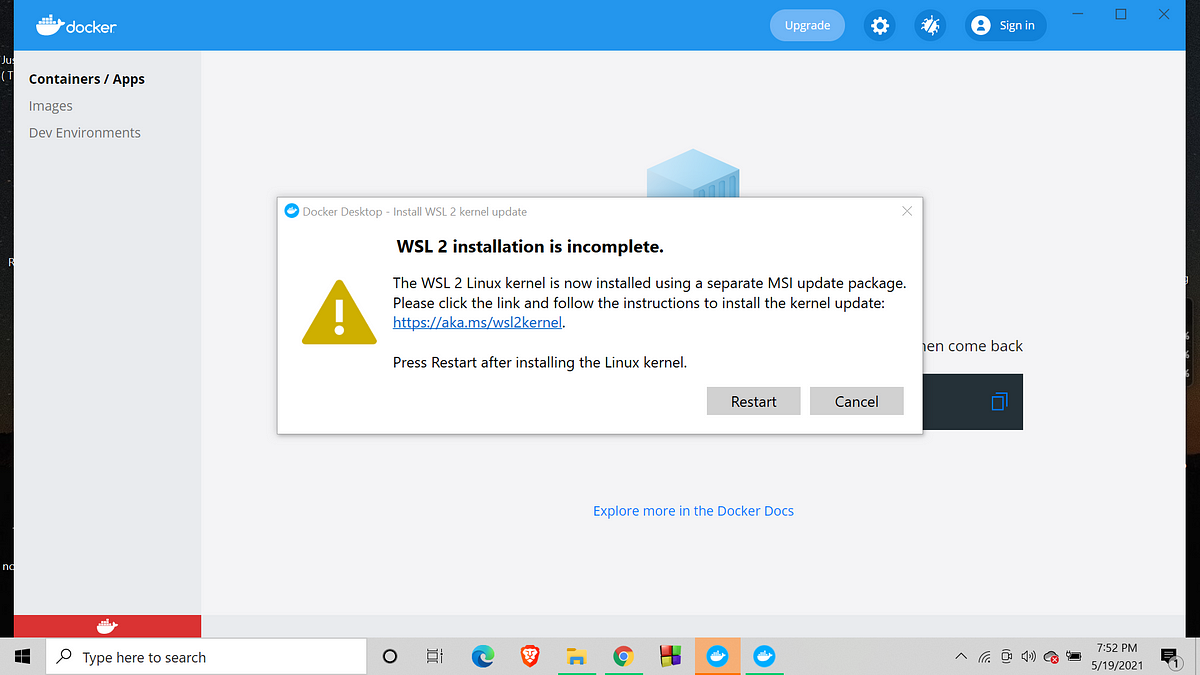The image shows a screenshot of a Docker webpage, featuring a light royal blue header with a large ship icon on the left and the word "docker" in all lowercase white letters. The header spans the top portion of the webpage, with a series of buttons aligned to the right, including "Upgrade," a gear icon for settings, a bug icon for troubleshooting, and a "Sign In" button. Additionally, the standard window controls—minimize, maximize/fullscreen, and close—are present.

Beneath this, the webpage has a sidebar on the left within a gray box containing navigation options labeled "Containers / Apps," "Images," and "Dev Environments." At the very bottom left of the sidebar, a red bar features the Docker ship icon once again.

In the main section of the webpage, there is a prominent warning message highlighted by a yellow triangle with an exclamation point. The message reads: "WSL 2 Installation is incomplete. The WSL 2 Linux kernel is now installed using a separate MSI Update package." Below the warning, there are two gray buttons offering the options to "Restart" or "Cancel."